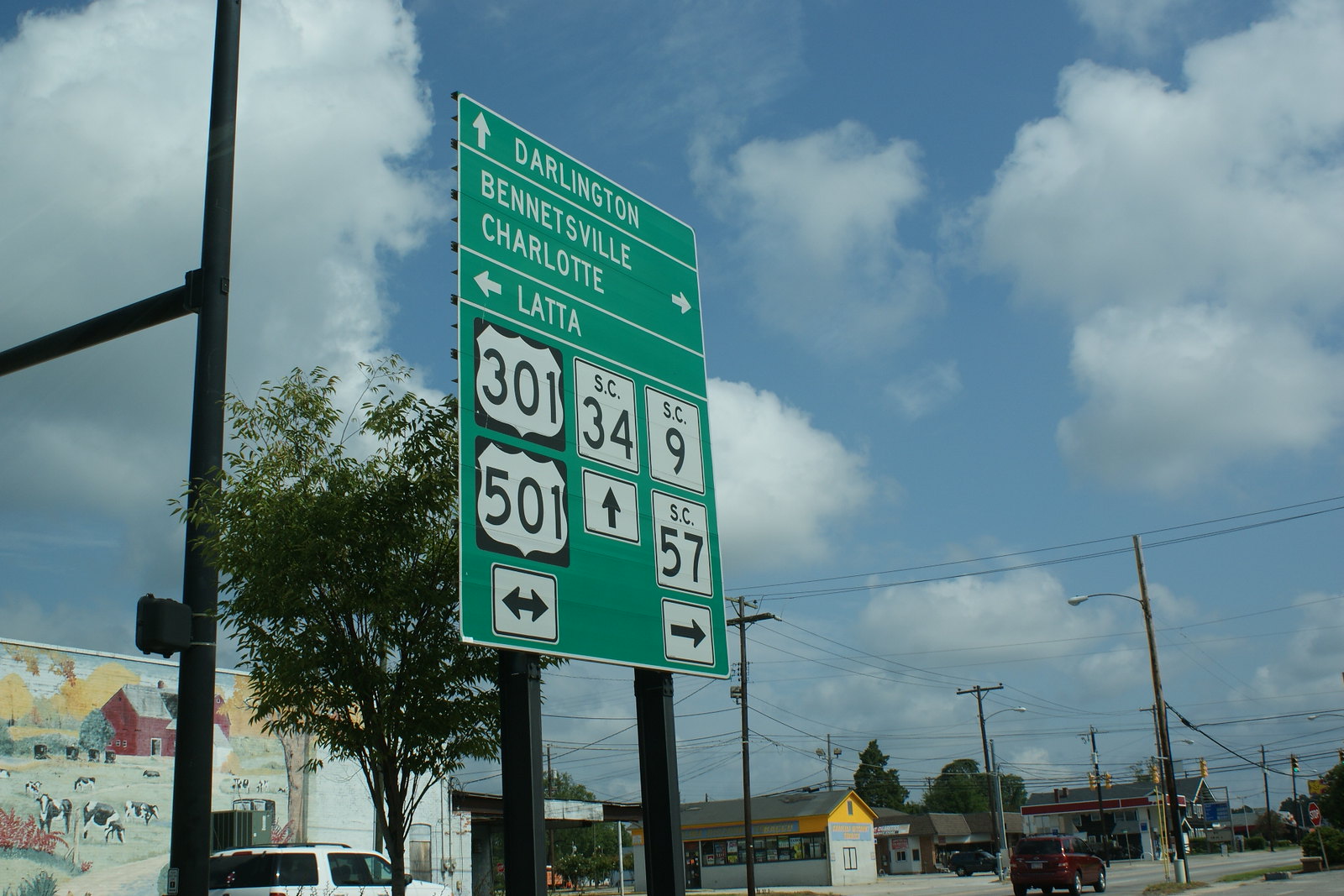This vivid photo, captured on a sunny afternoon, showcases a charming small town or rural area. The sky is a brilliant blue, dotted with numerous fluffy white clouds, creating a picturesque backdrop. In the foreground stands a prominent green road sign bordered in white, mounted on two black metal poles. The sign features multiple directional arrows: the top arrow points forward and indicates "Darlington," the second arrow points right towards "Bennettsville, Charlotte," and the third arrow points left towards "Lata" (spelled L-A-T-T-A). Below these arrows are several state route signs with additional arrows pointing left and right.

At ground level, there's a small convenience store visible, and across the street, a gas station can be seen. Numerous telephone poles with a web of telephone wires line the street, adding to the rural atmosphere. A small SUV is driving down the road, while a white station wagon is parked in front of a business on the left side of the photo. The scene is detailed, capturing the essence of everyday life in a quaint, small-town setting.